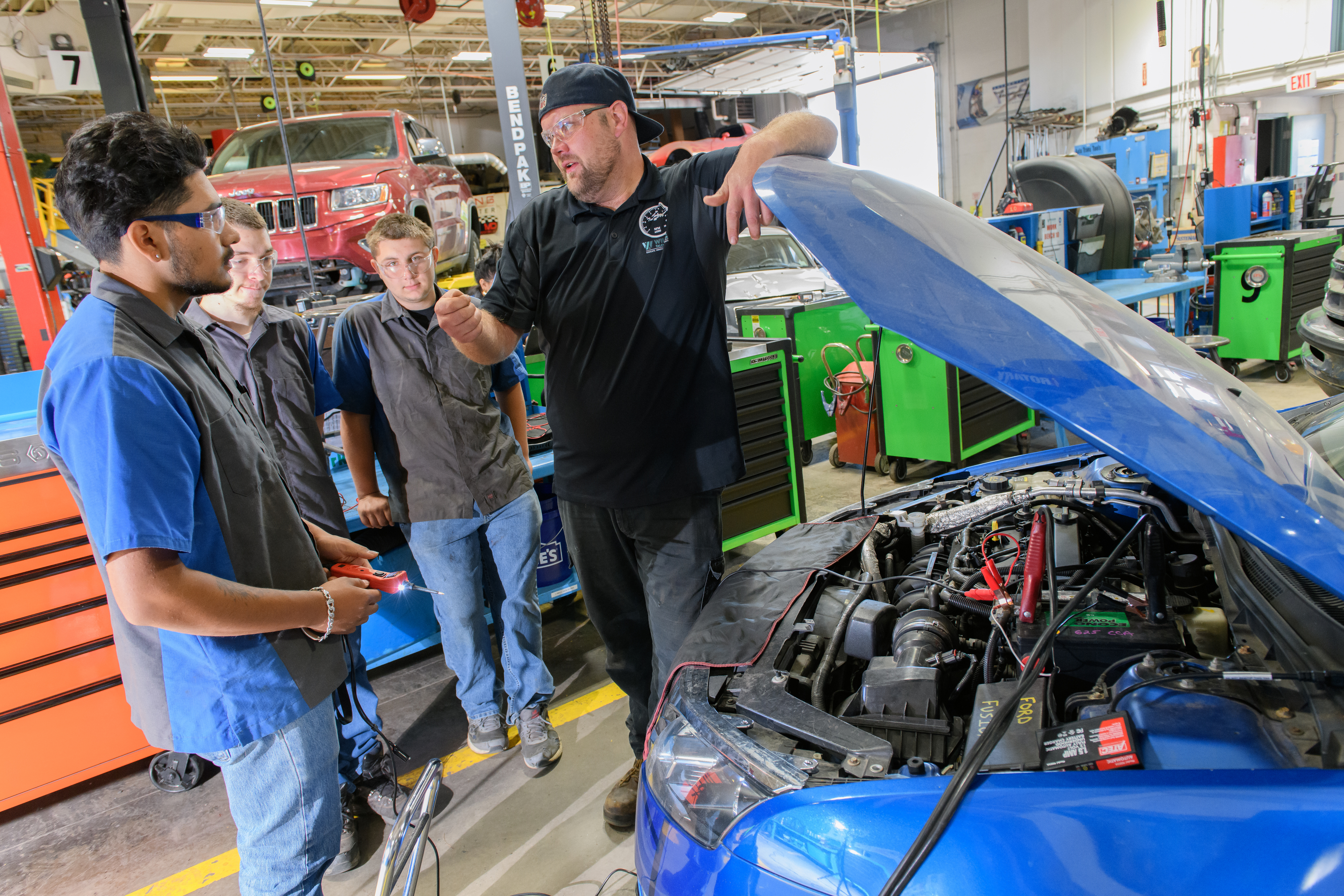The image depicts four men standing in what appears to be an auto shop, with a backdrop of various toolboxes and cars in different stages of repair. Positioned to the left, one man in a blue t-shirt with a black front and blue jeans, is holding a red tool with a light at its end, and wearing goggles. Next to him, two shorter men are dressed in black shirts and blue jeans, also wearing goggles. On the far right stands a man in all black clothing — black shirt, jeans, and boots — with a black hat worn backwards. His left arm rests against the raised hood of a blue car, seemingly explaining something to the others. The engine is visible, adorned with black, red, yellow, and green components, and jumper cables are attached to the battery. Behind them, the shop features light green cabinets and a variety of colorful toolboxes. Notably, a red SUV (or Jeep) is elevated on a lift, alongside other vehicles, including what appears to be a white car and possibly a Corvette, against the white walls of the well-lit garage. The clear, bright setting highlights the vibrant mix of colors throughout the scene.